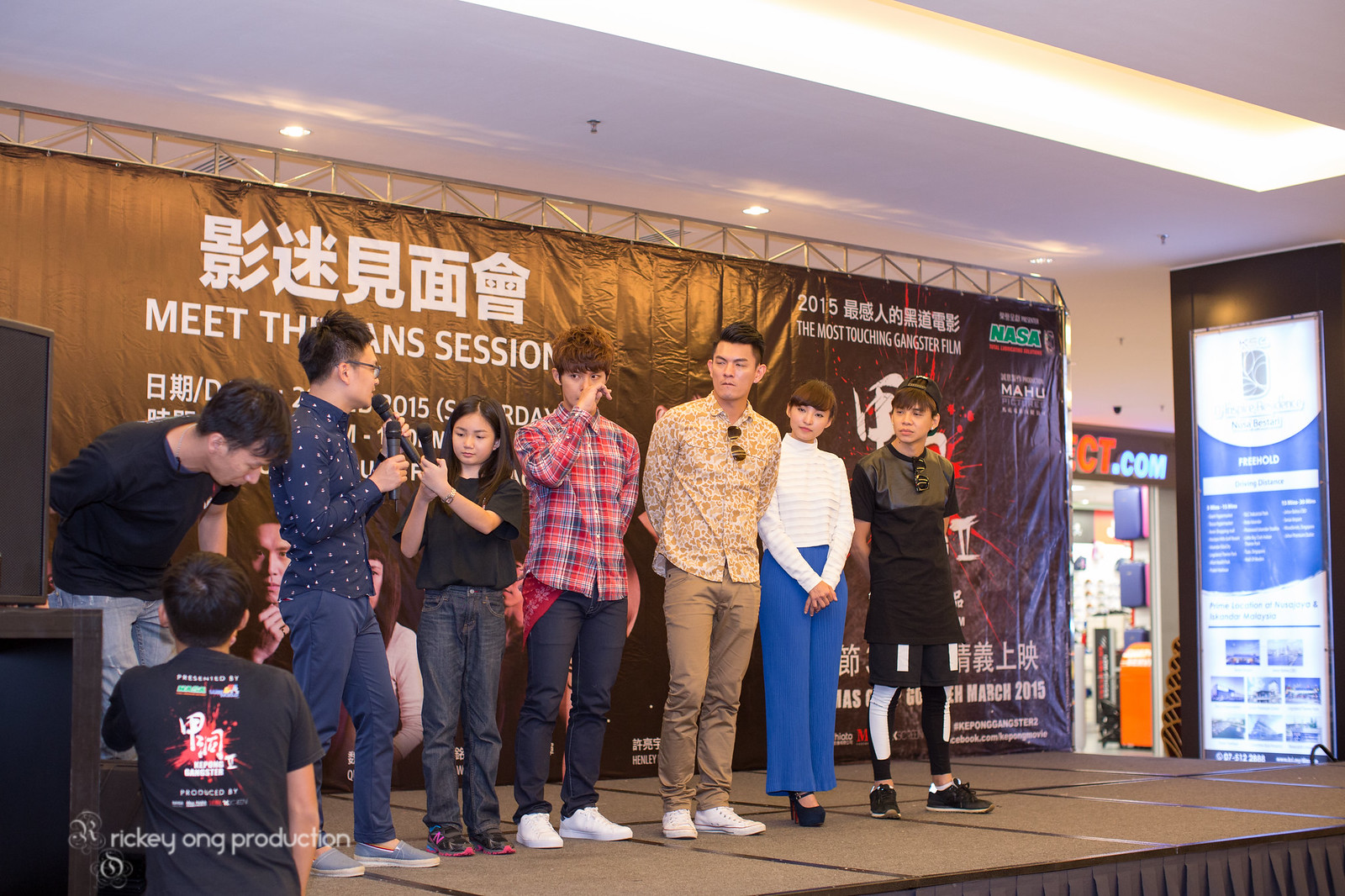In this color photograph, we see a group of approximately eight individuals of varying ages, predominantly Asian, standing on a black and gray stage within what appears to be a convention or meeting hall. The group comprises both adults and children, lined up from left to right with varying levels of attention directed towards the central figure. The man at the center wears a blue long-sleeved shirt with white spots, paired with blue pants. He holds two microphones, speaking into one while holding the other. Beside him, a middle school-aged girl in jeans, a black t-shirt, and sneakers stands quietly with her microphone poised but not in use. 

The stage itself is flanked by two sheets of banners. The top of the main brown banner features Asian script, subtitled by partially visible English text reading "meet the something session" likely obscured by the man's head. An address appears below this text. The second banner on the right side displays black with colored Asian lettering. Notably, in the bottom left corner of the image, text reads "Ricky on production." The ensemble further includes a young boy in a red shirt, another in a yellow shirt, and an adolescent in sporty attire complete with a backward hat.

A woman in blue pants and a dressy top, accompanied by a long-sleeved sweater, stands among them, alongside a man kneeling down as if to speak to someone off-stage. The environment is brightly lit with fluorescent lighting, and the style of the photograph is representational realism, capturing a candid moment in what seems to be an organized event or presentation session.